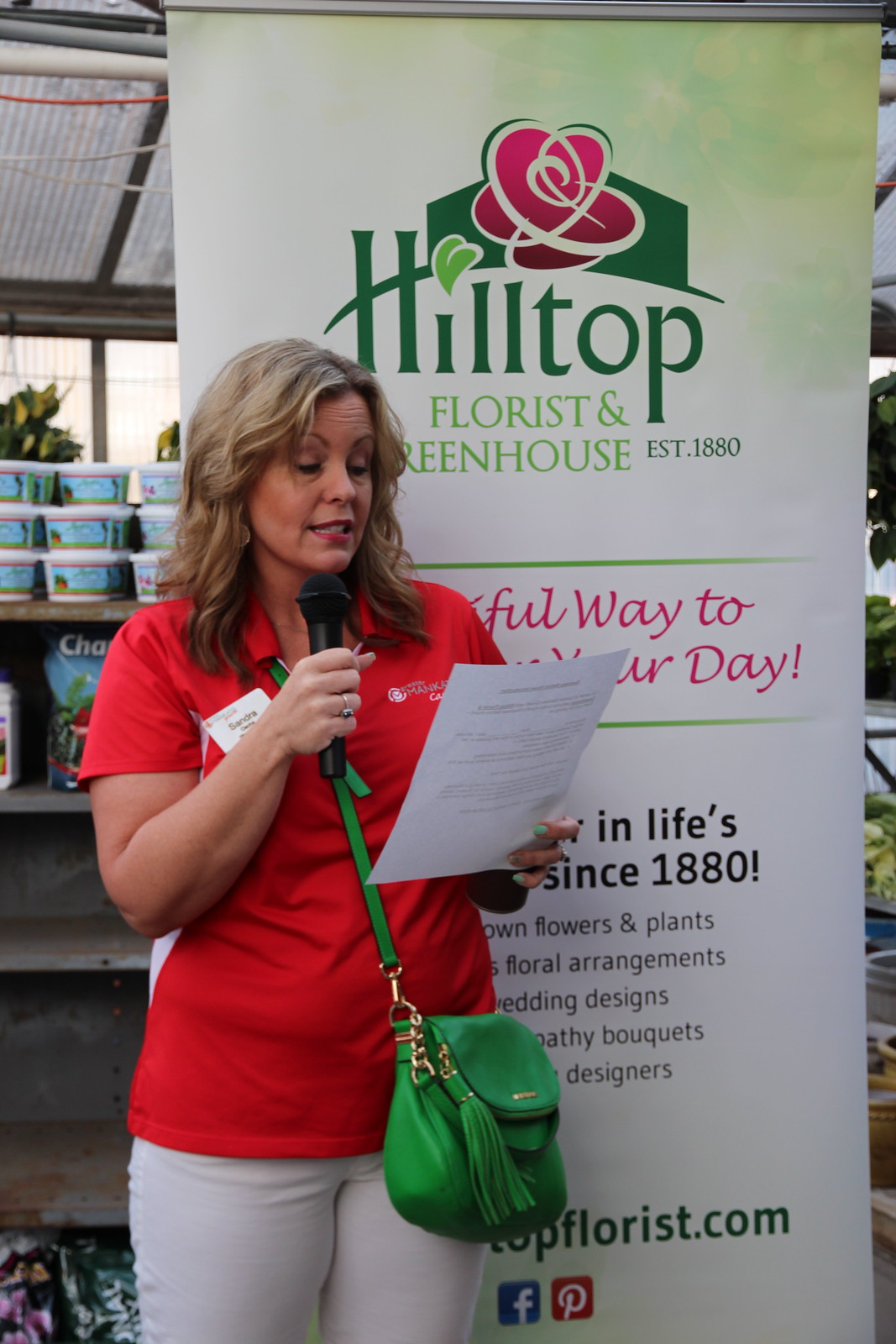In this outdoor or greenhouse setting, a middle-aged Caucasian woman named Sandra is captured in mid-speech, reading from a piece of paper while holding a microphone. She stands confidently in front of a large, white banner that reads "Hilltop Florist and Greenhouse, established 1880," though parts of the sign are obscured by her presence. The banner also features text promoting services such as "flowers and plants, floral arrangements, wedding designs, sympathy bouquets, designers," and shows icons for Facebook and Pinterest.

Sandra’s wavy blonde hair frames her face, which is accented with makeup. She wears a red polo shirt with a name tag that reads "Sandra," and pairs it with white pants. Draped across her body is a green crossbody purse adorned with a small tassel. Adding a touch of elegance, she has a ring on the ring finger of her right hand. Behind her, one can glimpse bags of potting soil, flowers, tubs, plastic containers, and other gardening products, lending a busy and industrious atmosphere to the scene.